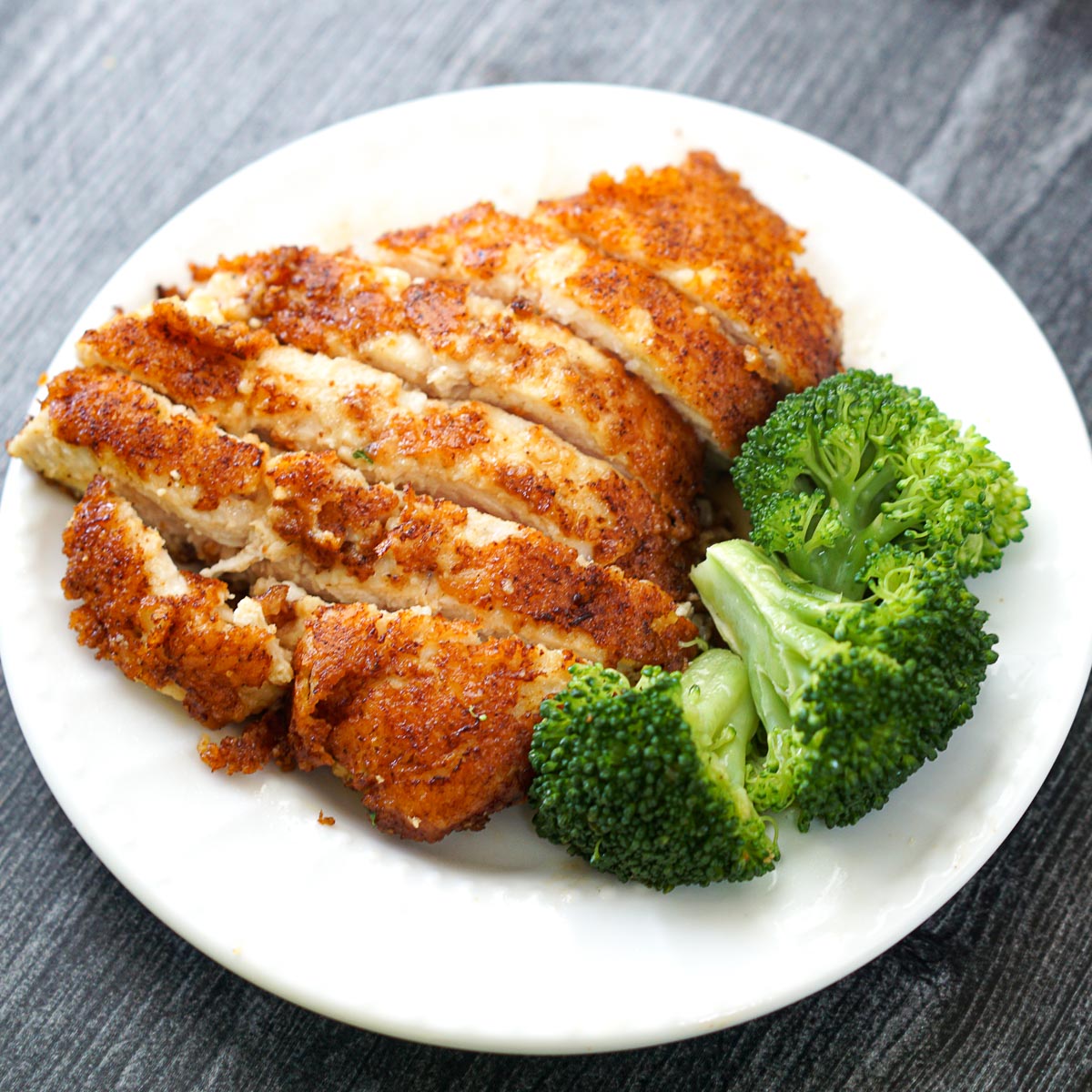This indoor photograph captures a close-up of a plate of food presented on a gray-stained faux wood table with a grain running diagonally from the lower left to the upper right. The circular white ceramic plate is slightly angled and partially extends out of the frame on both the left and right sides. On the right side of the plate are three vibrant, steamed broccoli florets with stalks, adding a bright green contrast. On the left side rests a succulent portion of breaded fried chicken breast, which has been sliced into thin, horizontal strips. The chicken appears tantalizing with its light to dark brown breading, glistening from oil. Above the plate, a light source illuminates the scene, causing a mild blur in the upper left corner of the image, enriching the texture and detail of the meal.